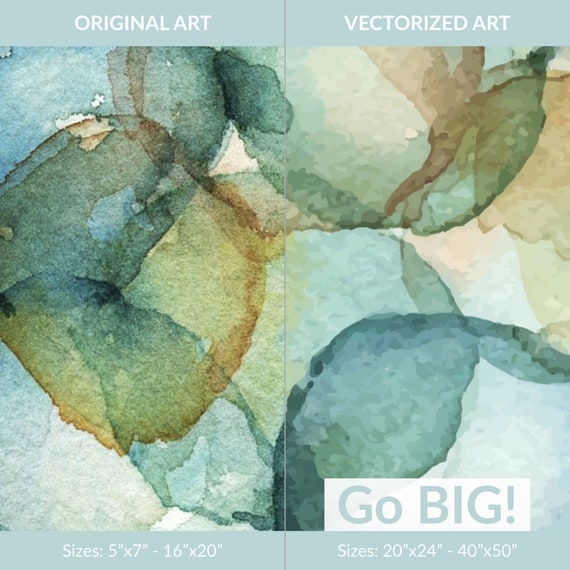The image is a split-screen digital illustration comparing original art on the left with vectorized art on the right. Both halves are dominated by abstract shapes in various shades of green, light blue, and white, set against a light blue background. Each side is labeled at the top in a light blue rectangle with white text; the left side reads "Original Art," and the right side reads "Vectorized Art." The left side also includes text in a light blue rectangle at the bottom that indicates the sizes available: "5 by 7 inches to 16 by 20 inches." The right side features larger sizes, labeled "20 by 24 inches to 40 by 50 inches" in a corresponding light blue rectangle at the bottom. Above this, a white rectangle with green text boldly states, "GO BIG!" The abstract shapes in the illustration resemble organic forms, almost like fish, and are composed in a manner that suggests fluidity and movement, enhanced by the pastel and turquoise hues.